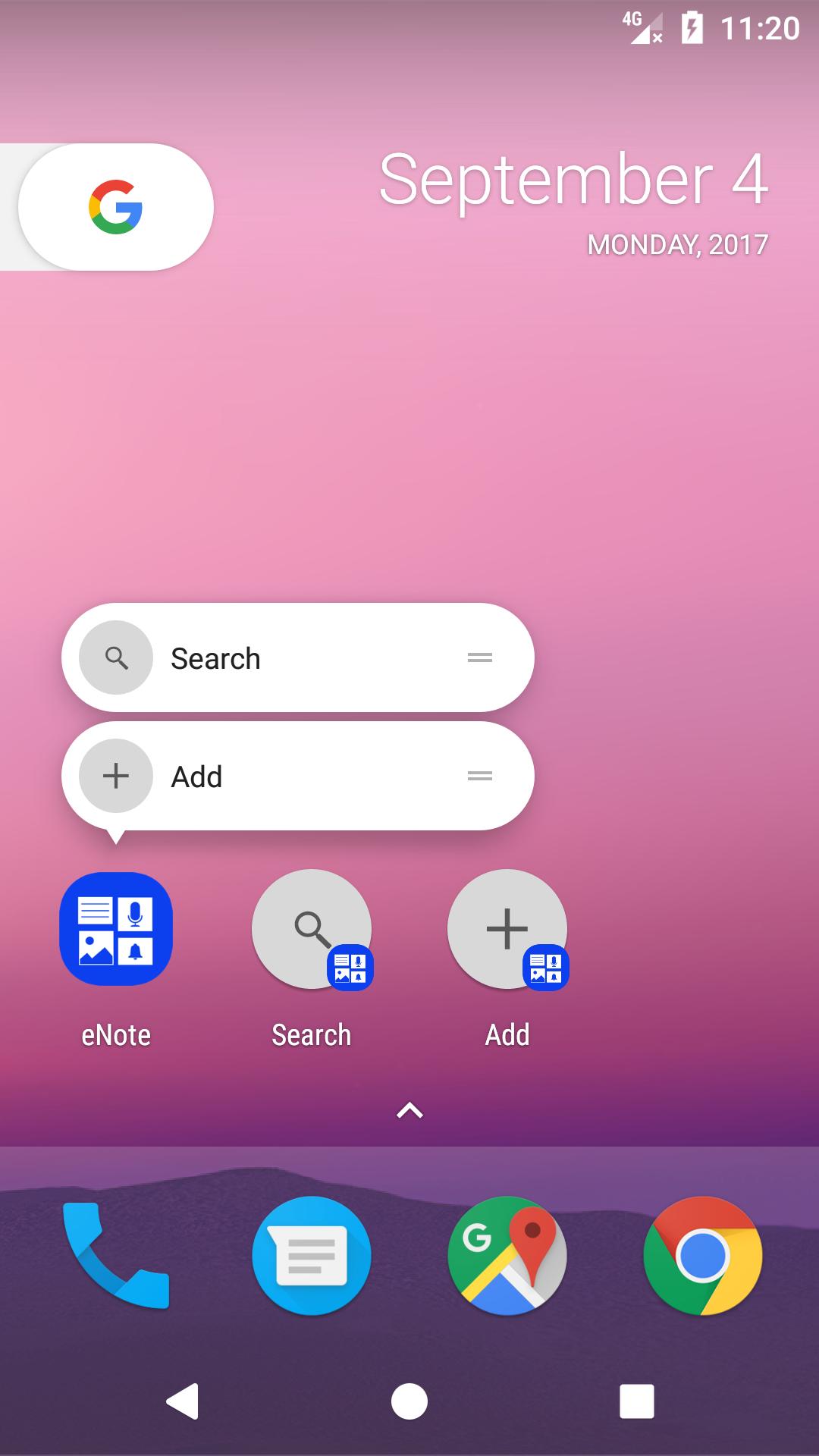This image is a vertical screenshot captured on a mobile device, prominently featuring a minimalistic and gradient-themed background. The gradient starts with a darker pinkish-purple hue at the top and bottom, gradually becoming lighter towards the middle. Near the bottom of the image, there's a simple depiction of a shale gray mountain edge, contrasted by a lavender-colored body of water below it.

At the top of the screenshot, the time is shown as 11:20, along with an indicator that the battery is fully charged and currently charging. Below this, in white text, the date is displayed as "Monday, September 4, 2017."

On the left side of the screen, there's a slider with the Google "G" logo. Below it, there's a search bar that contains the word "Search" accompanied by a magnifying glass icon. Underneath the search bar, another text bubble reads "Add," which includes a grey circle with a plus sign inside it. Additionally, there are three app options listed:

1. "e-note,"
2. "Search," each accompanied by blueish squares with rounded edges bearing different icons,
3. "Add."

At the bottom of the screen, four icons are arranged in a row:
- A blue telephone icon,
- A blue chat messenger bubble icon,
- The Google Maps icon,
- The Google Chrome icon.

This detailed screenshot provides a clear view of the mobile interface, highlighting its functional and aesthetic elements.